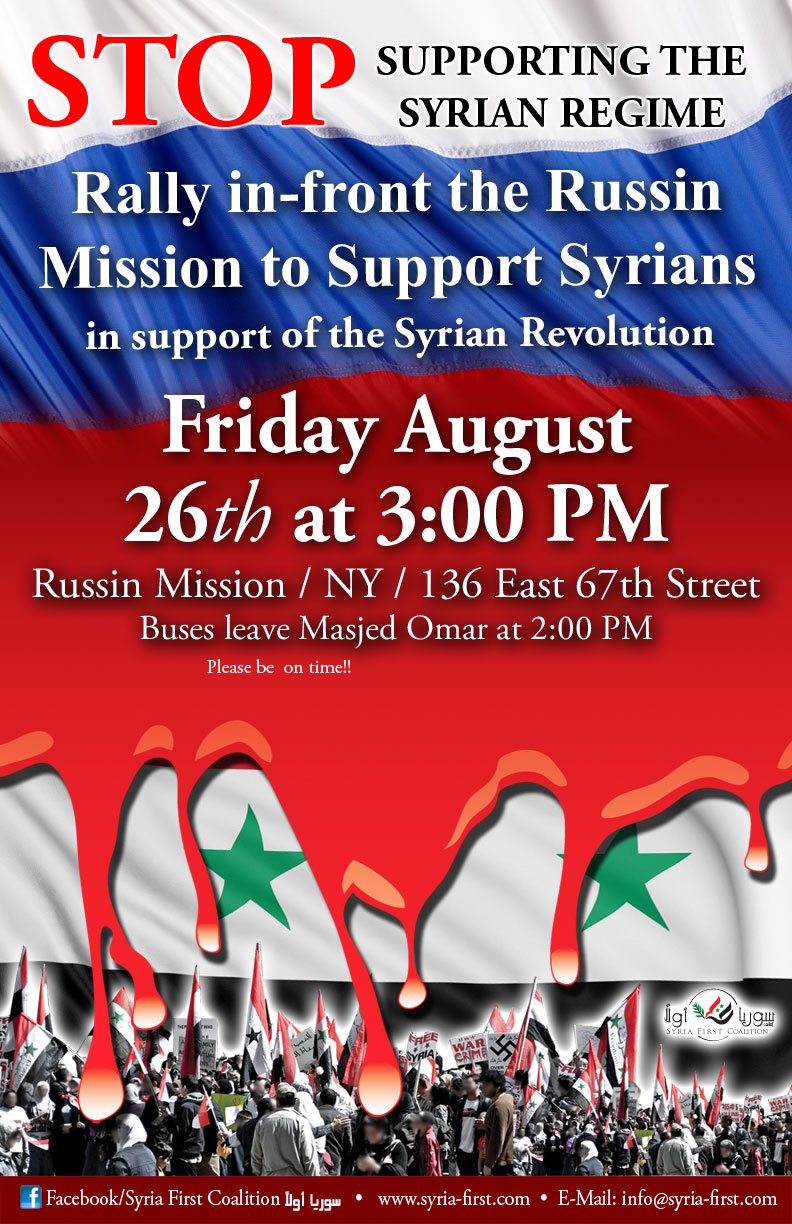The image depicts a detailed flyer for an event protesting the support of the Syrian regime. Dominating the design is a background featuring the Russian flag, with red at the bottom dripping like blood onto a white section adorned with green stars. Above, red text demands "STOP," followed by "supporting the Syrian regime" in black. Below the dripping flag imagery, there's a crowd of people holding Syrian flags and banners, including one bearing a swastika, suggesting the event is a demonstration or protest. The flyer provides information about a rally titled "Rally in front of the Russian Mission to support Syrians in support of the Syrian Revolution." The event is scheduled for Friday, August 26th at 3pm, located at 136 East 67th Street, New York. Buses will depart from Masjid Omar at 2pm, with a note urging attendees to be punctual. The bottom of the flyer includes contact information with the Facebook handle "Syria First Coalition," the website "www.syriafirst.com," and an email address "info@syriafirst.com."